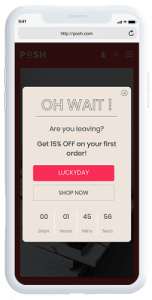Detailed Caption:

An iPhone is prominently displayed in the image, showcasing an open webpage. The status bar at the top indicates the time as 9:41, a full battery, and a strong Wi-Fi connection. The URL in the address bar is partially visible, starting with "https://," though the rest of the website name appears blurred, possibly resembling "posh.com." A refresh icon is also present in the address bar.

Dominating the middle of the screen is a common pop-up box frequently encountered on retail websites. This pop-up, intended to prevent the user from leaving the website, features a persuasive message stating, "Wait, are you leaving? Get 15% off on your first order! Lucky day! Shop now.” Below this message, a clickable button labeled "Shop Now" encourages immediate action.

At the bottom of the pop-up, a countdown timer is displayed, detailing the remaining time to claim the offered discount. The timer shows "1 hour 45 minutes and 56 seconds" remaining for the user to take advantage of the 15% discount. Clicking the "X" at the top of the pop-up would close the box, returning the screen to its regular state, no longer grayed out by the overlay.